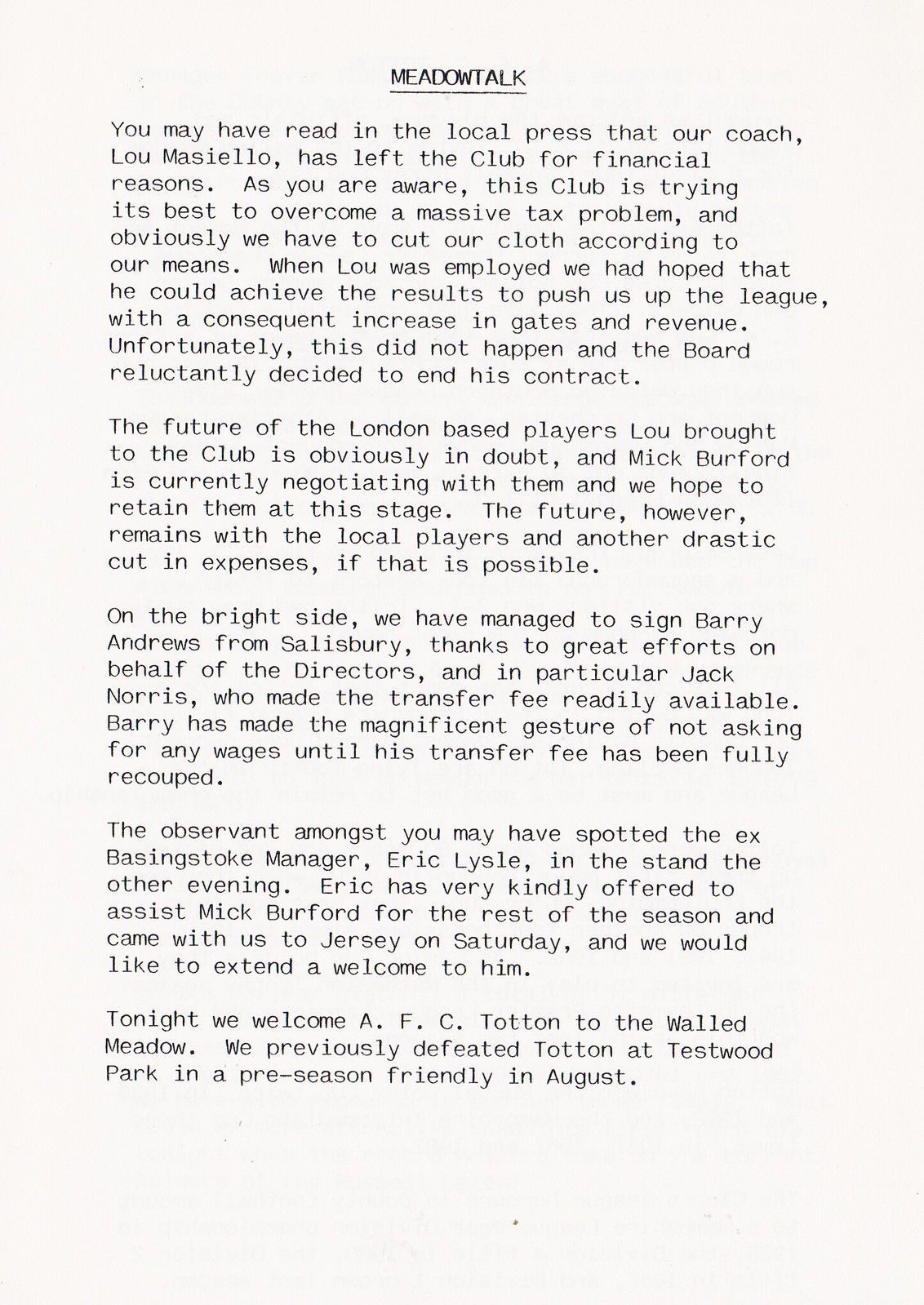The image displays a tan-colored printed piece of paper featuring multiple lines of black text. At the very top center of the paper, the title "METALTALK" is prominently underlined and capitalized. Below the title, the text is organized into several paragraphs. The document starts by addressing the readers about recent changes in the club, mentioning that the coach, Luis Macielo, has departed due to financial reasons amidst the club's struggles with a significant tax issue. The narrative explains that while the coach was initially employed to boost the team's league position without affecting revenue, these results were not achieved, leading to the termination of his contract. The future of the London-based players brought in by Macielo is now uncertain, with Mick Burford negotiating their positions. The article emphasizes that the team will continue mainly with local players and hints at further developments. Additionally, the last paragraph expresses a welcoming note to AFC Taunton for a match at Walled Meadow, recalling a previous preseason friendly victory against Taunton at Testwood Park in August.